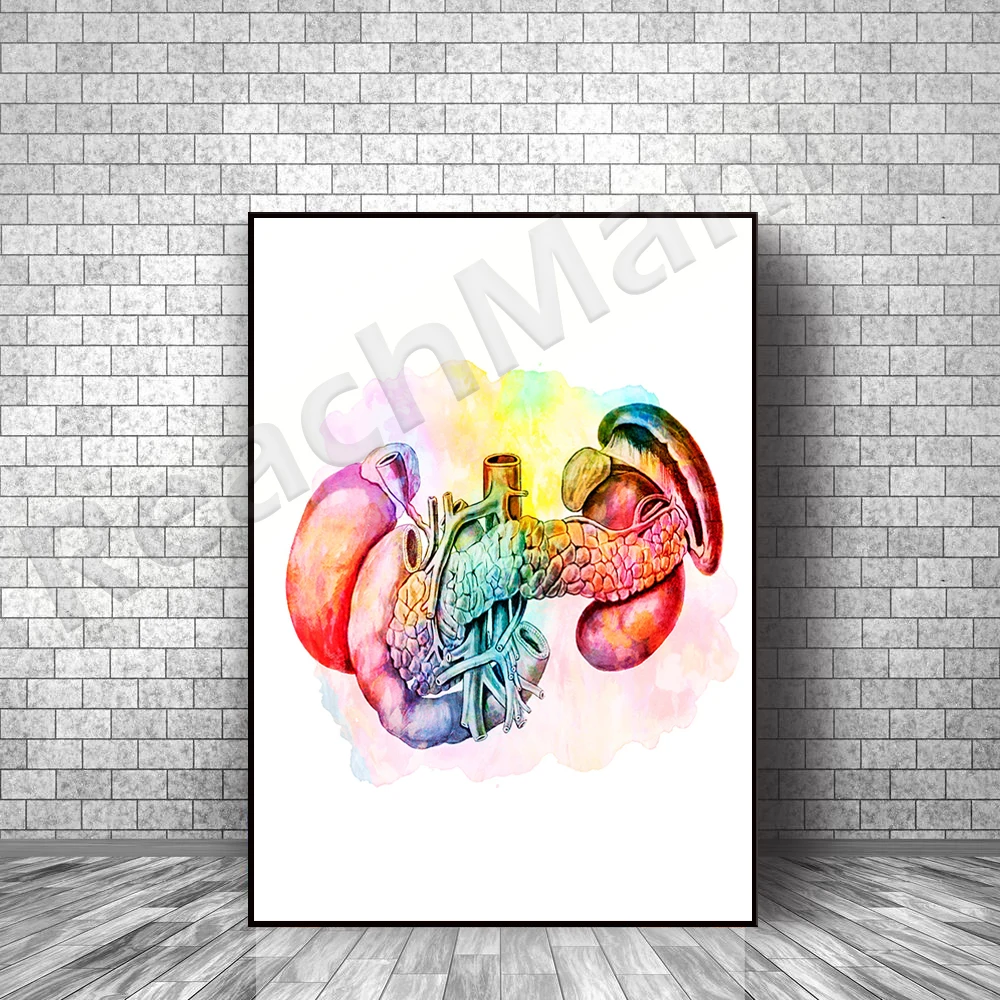This detailed drawing illustrates a collection of human internal organs, prominently displayed against a stark white backdrop. The composition, set against a textured gray brick wall that features alternating shades of lighter and darker gray, adds a contrasting rugged charm to the scene. The floor, echoing the gray palette, is laid out in a pattern reminiscent of wooden flooring, providing a sophisticated tiled appearance. Centrally positioned, the anatomical depiction highlights various organs, predominantly colored in shades of red with bluish tints towards their core. The identifiable organs appear to include the kidneys, intestines, and potentially the spleen, among others. Adding an intriguing layer to the image, a piece of text reading "REACHMANI" stretches diagonally across from the lower left to the upper right, further emphasizing the focal point and inviting curiosity.